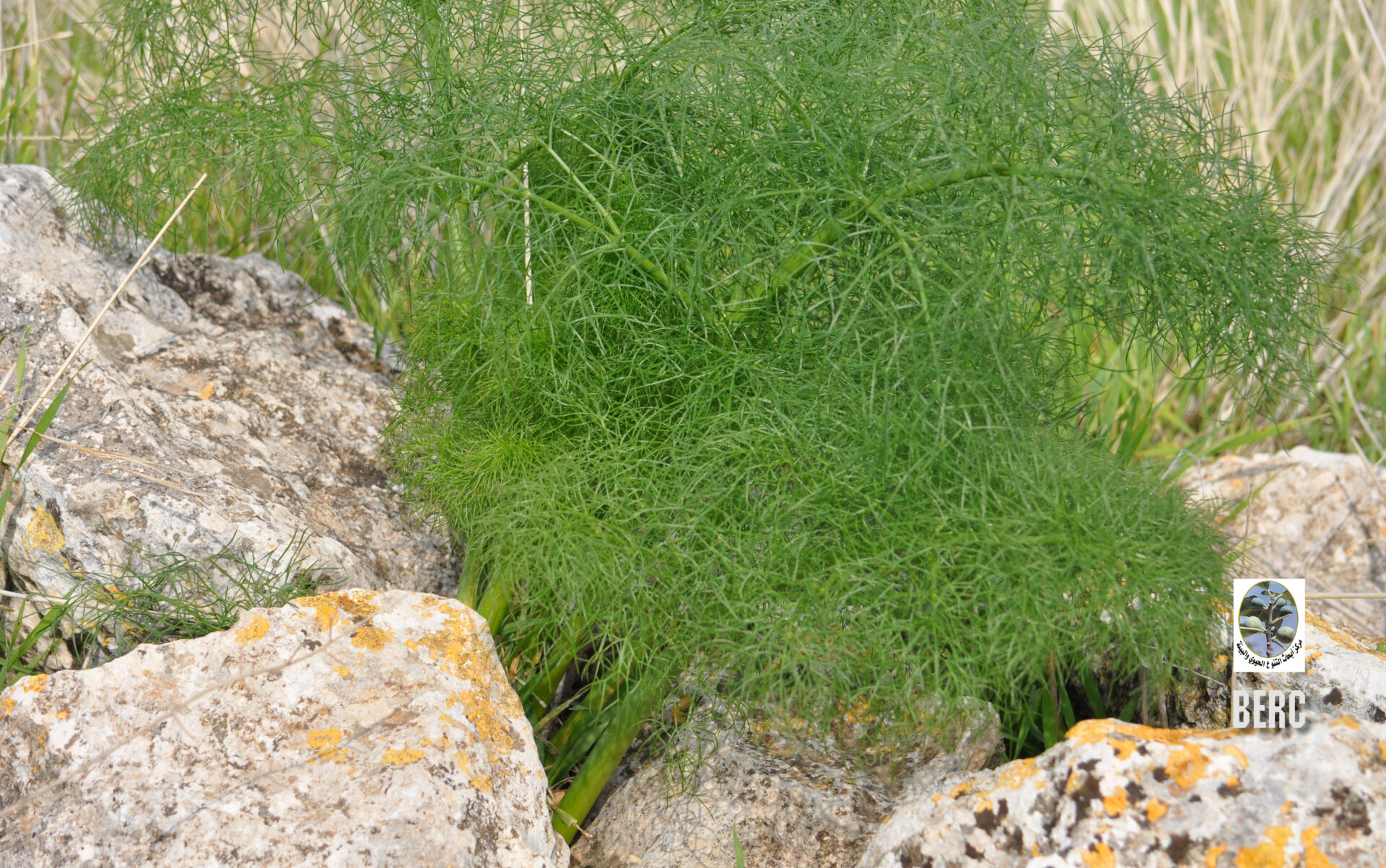This daytime outdoor photo captures a detailed and vibrant scene of nature. In the image, several large boulders dominate the foreground, stretching from the right-hand side towards the left. These boulders, which are a mix of granite and other types of rock, exhibit a range of hues including gray, brown, and yellow, with patches of white, black, and yellow moss and lichen adding texture. Nestled in the cracks between these rocks, a wild green plant grows, its thin, delicate leaves resembling those of fennel, dill, or parsley. In the background, long, overgrown brown grasses and bushes create a natural backdrop. The overall composition frames the natural harmony between rocks and plant life, with the lower right-hand corner featuring the subtle lettering "B-E-R-C."